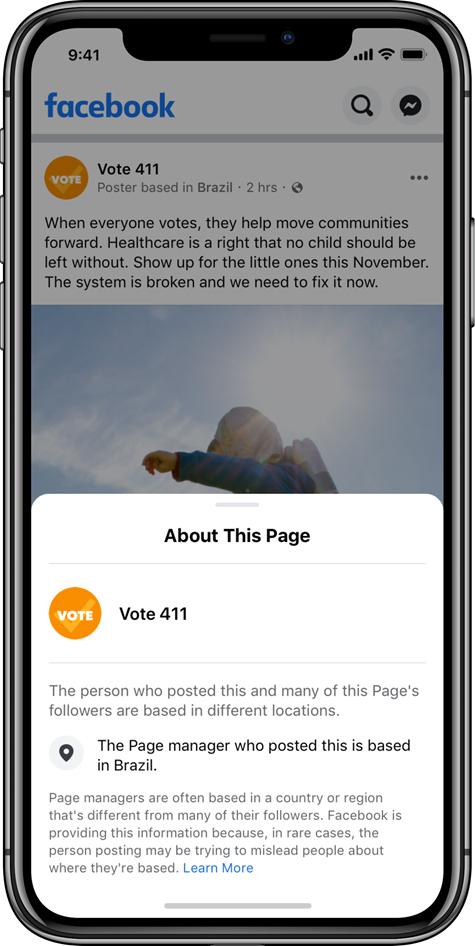A blackish-gray bezel iPhone is displayed against a white background with a gray overlay. On the left side of the device, near the top, there's a small button followed by two larger ones below it. The right side features a single button aligned with the second and third buttons on the left. The screen showcases a central cutout for the front camera. At the top of the screen in black text, "9:41" is visible. To the right of the time display, icons indicate full cell signal strength, Wi-Fi connectivity, and battery percentage.

Below the top bar, the Facebook app is open, displaying its interface in blue. On the right, a black magnifying glass icon and the Facebook messaging icon are present. An orange circle with a white checkmark and the word "VOTE" draws attention. Next to it, "4/11" is written in black, indicating the post count. The post header reads in gray text, "Posted 2 hours ago in Venezuela."

The content of the post states: "When everyone votes, they help move communities forward. Healthcare is a right, and no child should be left without. Show up for the little ones this November. The system is broken, and we need to fix it now." Below this message, there is an image of a child set against a blue background. The post notes that the page manager is based in Brazil, revealing an effort to influence U.S. elections from outside the country.